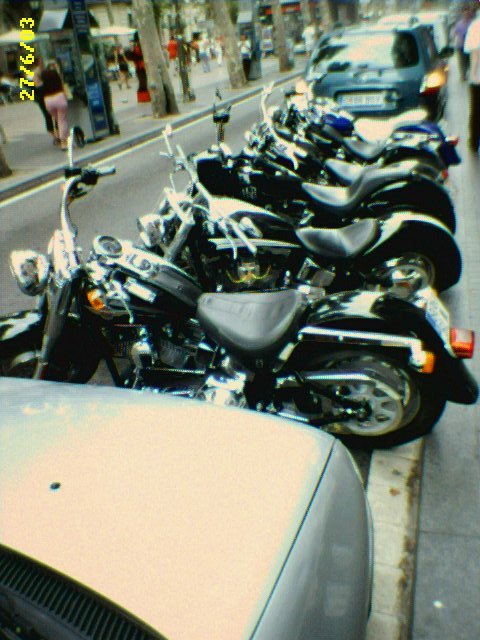The color photograph, likely taken on June 27, 2003 (indicated by the yellow timestamp in the top left corner), captures a bustling outdoor scene in what appears to be a European city. The image, slightly blurry and out-of-focus, showcases a narrow street flanked by wide sidewalks lined with trees and kiosks. 

At the center of the photo, a row of six neatly parked motorcycles, predominantly black in color and of a larger model, are wedged between two cars along the curb. Each motorcycle points outward towards the street, giving a clear and organized look to the parking arrangement. The street is busy with casually dressed pedestrians walking up and down the wide sidewalks, providing a lively atmosphere to the scene. The photograph has a dated aesthetic, complemented by the slightly worn appearance and potential filter effect, evoking a sense of nostalgia.